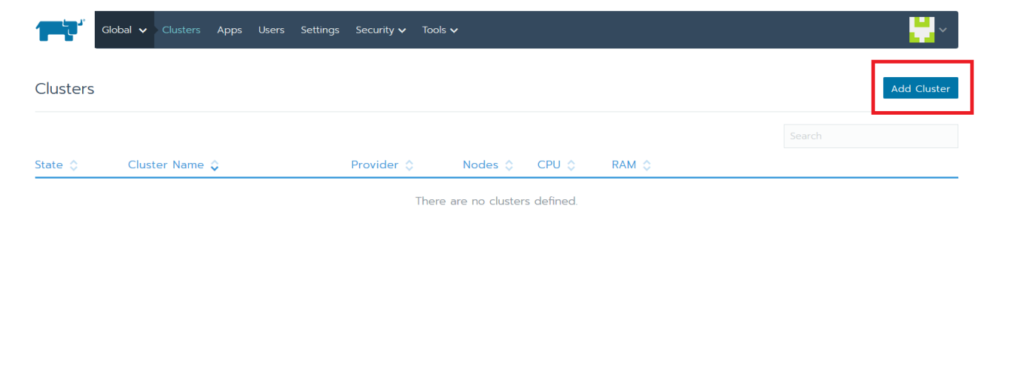Screenshot of a website interface. The image quality is low, appearing blurry and small. In the upper left corner, there's a blue icon of a cartoon bull, depicted with horns and facing right. Adjacent to this icon is a dark purple navigation bar featuring white text. The bar includes the following menu items: "Global," "Clusters," "Apps," "Users," "Settings," and "Security," each acting as drop-down menus. Additionally, there's a "Tools" drop-down menu. 

In the upper right corner, a profile picture placeholder is visible, represented by a white square with yellow dots. Below this placeholder, a prominent blue button with white text is highlighted by a red square outline, reading "Add Cluster." On the left side of the web page, "Clusters" is written in black font. Beneath this title, a thin black line separates it from a section header that lists "State," "Cluster Name," "Provider," "Node," "CPU," and "RAM" in blue text.